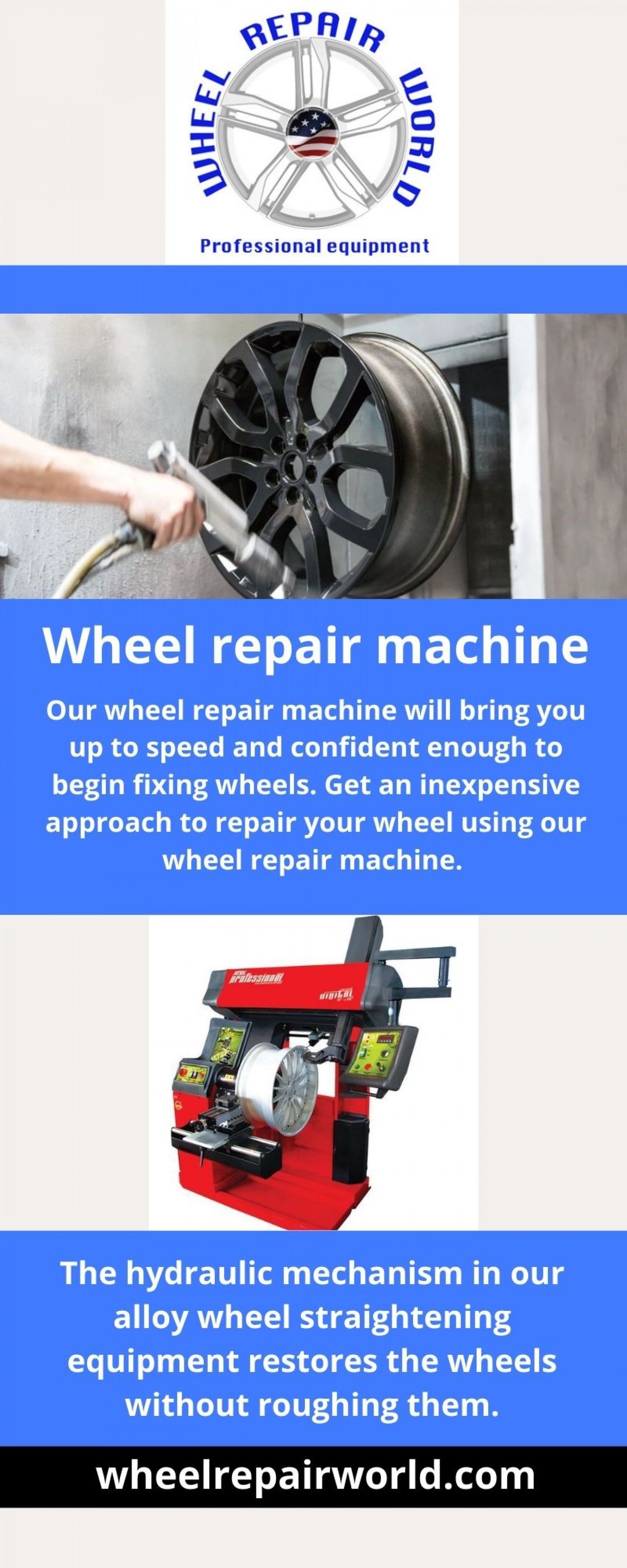This detailed advertisement for Wheel Repair World, presented in a tall, narrow pamphlet format, combines color photography, graphic design, and typography. Starting at the top, it features a logo depicting a silver wheel with an American flag hub, bordered by the text "WHEEL REPAIR WORLD" in blue, all caps. Below the logo is the subtitle "PROFESSIONAL EQUIPMENT." 

The main body starts with a blue stripe, followed by a landscape photograph showing a person's hand holding a paint sprayer working on a blue-black wheel hub. Underneath this image, a blue textbox with white text declares "WHEEL REPAIR MACHINE." 

A paragraph below explains that their wheel repair machine will boost your confidence and speed in wheel repairs, offering an inexpensive solution. Further down, a photograph shows a red machine with a mounted steel wheel. Another blue textbox details the hydraulic mechanism in their alloy wheel straightening equipment, emphasizing its gentle yet precise performance. 

At the very bottom, a black strip with white text directs readers to visit "wheelrepairworld.com" for more information about their services and equipment.